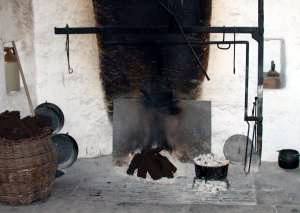This is an indoor scene, possibly reminiscent of pioneer times, captured in a color photograph of what appears to be a living room or another central room of a small dwelling. The room is encased by whitewashed stone or stucco walls with a fireplace in the center, which shows signs of burning. A metal bar hangs above the hearth, suggesting it is used for cooking, with associated metal implements around. A wooden barrel sits on the left, accompanied by shallow wooden pans and additional black cooking tools. Adjacent to this is a tall dark wicker basket and a white and brown jug on a nearby shelf. The floor is constructed from gray stone, featuring a black metal pot filled with a white substance and standing on legs. Another black pot rests on the far right, near a large metal plate leaning against the wall. The right side of the image also shows a post with a horizontal extension, from which objects hang.